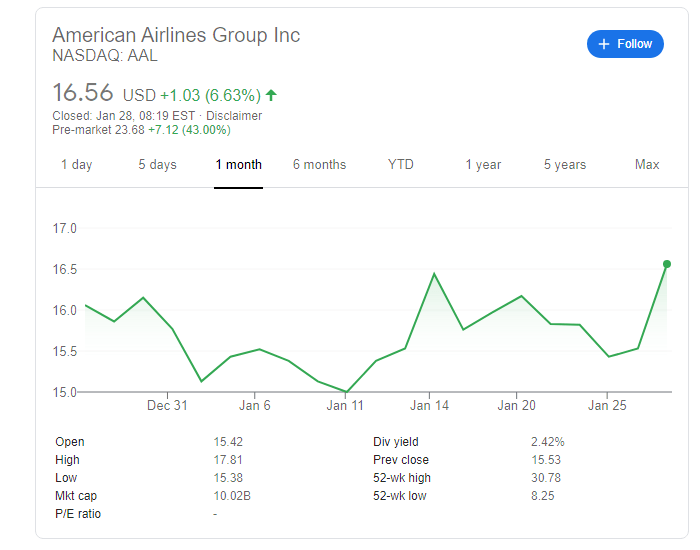The image depicts a computer screen displaying a stock information interface for American Airlines Group Incorporated. In the top-left corner of the white rectangle, the text reads "American Airlines Group Incorporated" with "NASDAQ: AAL" directly below it. In the top-right corner, there is a blue-colored button labeled "+ Follow," allowing users to opt-in for updates.

Beneath this heading, the current stock price is shown as "16.56 USD," accompanied by a change indicator of "+1.03" and a percentage increase of "(6.63%)" with an upward arrow, signifying a rise in the stock value.

Below the stock information, a line graph visualizes the stock's performance over time. The vertical axis, situated on the left side, is marked with price points starting at 15.0 and incrementing through 15.5, 16.0, 16.5, up to 17.0. The horizontal axis at the bottom of the graph is labeled with dates: December 31st, January 6th, January 11th, January 14th, January 20th, and January 25th.

The line graph itself traces the stock’s movement, beginning at 16.0 and ending at 16.5, with a noticeable dip in the middle before it ascends again, reflecting fluctuations in the stock's price over the specified period.